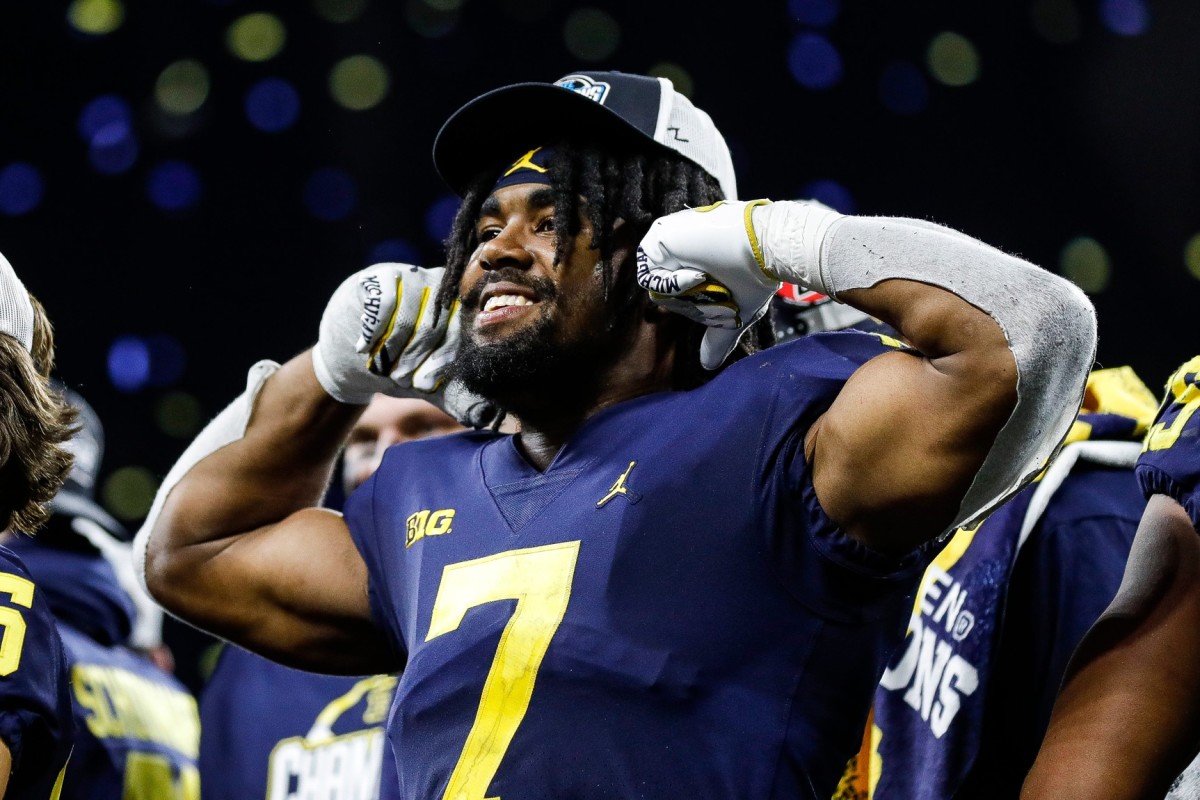This nighttime outdoor photograph captures a jubilant football player of African descent at the center, wearing a dark blue Michigan Wolverines jersey with the number seven in bright yellow and a "Big Ten" patch. His intense celebration is shown by his muscular arms raised towards his face, with white gloves on his hands and his fingers seemingly plugging his ears as he grins broadly, revealing his white teeth. He sports a black and white trucker hat over a black headband adorned with a gold Air Jordan logo, contrasting against his black ringlet hair and full beard. His uniform includes white arm sleeves extending from beneath his jersey. Surrounding him, other team members in matching gear are visible, though their faces are obscured, underscoring his central joyful presence against a backdrop dotted with out-of-focus gold and blue lights, adding to the festive atmosphere of the scene.